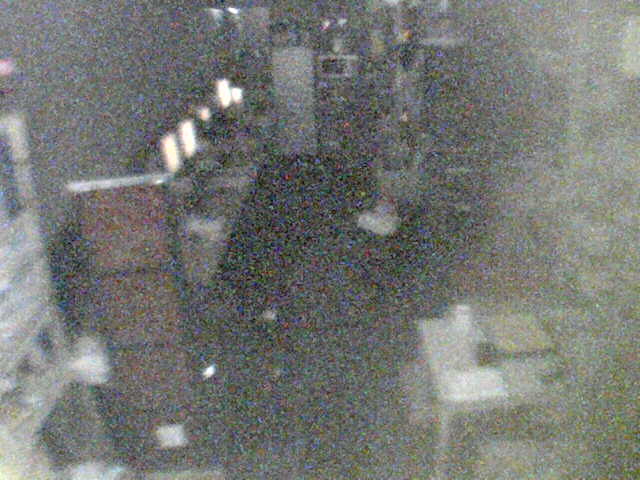This extremely fuzzy and grainy photograph, possibly taken from a security camera high up on a wall, depicts a room that is difficult to clearly identify due to the poor image quality marked by blue, green, and red speckling. On the left side of the room, there are multiple glowing screens, likely computer monitors or open laptops, aligned with a desk that stretches in front of them. Behind this desk area, there is a gray wall leading to a white door. In the far background, there might be a white refrigerator and a small microwave placed on a shelf. Midway along the left wall, plastic shelves holding various items are visible. To the right, a table appears to hold a coffee cup, napkins, and assorted objects. The room might be a break room, storage area, or possibly even a kitchen, although the items within suggest it’s not a retail space.